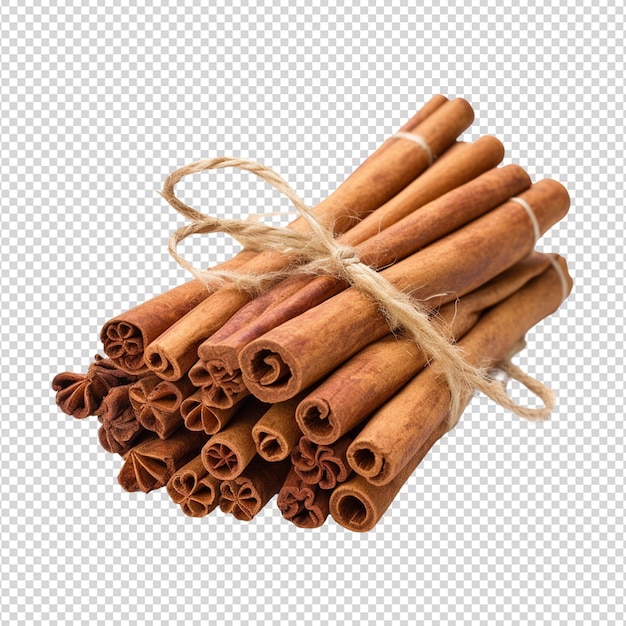This image depicts a simple yet intriguing bundle of approximately 15 to 20 cinnamon sticks, each about 4 to 5 inches long, tied together with a piece of tan, rough twine in the center, forming a bow with the loops facing left. The cinnamon sticks are cylindrical and exhibit varying thicknesses but are of uniform length, held together in a tight bundle. 

At the top ends of the sticks, some display intricate, decorative carvings—featuring floral patterns, triangles, moons, and circles—while others retain their natural spiral form. Additionally, a few sticks have a white elastic band around their far ends, adding a unique contrast to the overall appearance.

The background is a repeating pattern of gray and white checkered squares, indicating that the image might have a transparent background suitable for overlays. The entire composition is in sharp focus, presenting a clear and detailed view of the cinnamon sticks' texture and color, which is a rich brownish-orange. The minimalist and transparent nature of the backdrop accentuates the cinnamon sticks, making them the focal point of this stock photograph.